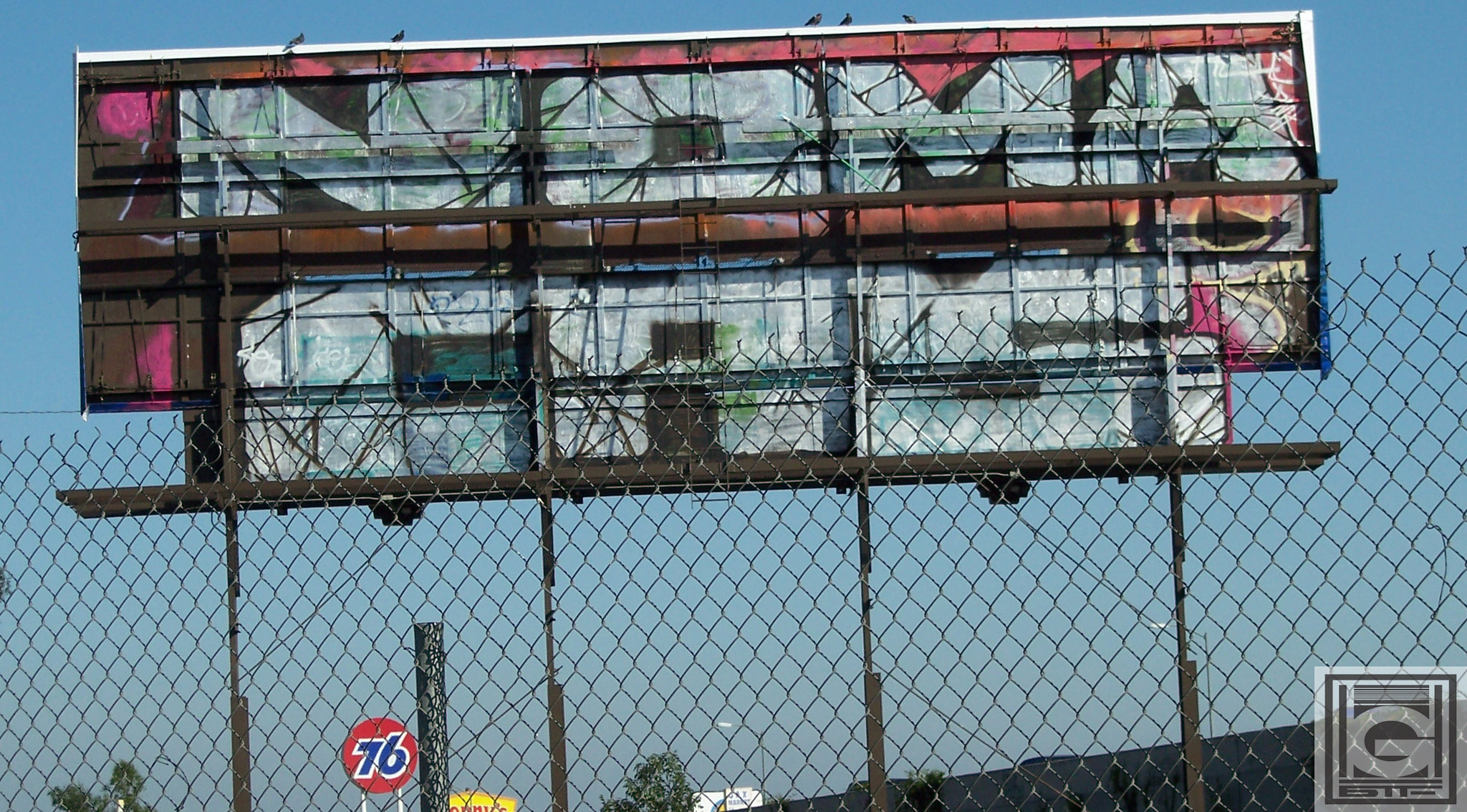In the image, the bottom right corner prominently features a large, stylized letter 'G' accompanied by some text. In the foreground, there is a chain-link fence with rustic wooden poles, which adds a gritty feel to the scene. The background is dominated by a vibrant orange circle displaying the blue number '76'. Above this circle is a yellow sign for 'Denny's'. To the side, a lush green tree adds a touch of nature. Towering over everything is a grand billboard that seems to have 'Nomakash' painted on it in graffiti-style, purple bubble letters. The lettering is outlined in red and has a white border, giving it a dynamic, multi-colored appearance.